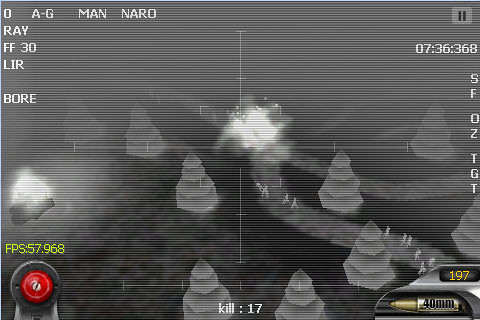This image appears to be a screenshot from a video game. Dominated by a predominantly gray color scheme, the focal point is a thin white crosshair in the center, resembling a plus sign with four lines that do not intersect at the middle. To the left, a conspicuous red button is visible. At the bottom center of the screen, the word "Kill" is prominently displayed, accompanied by a kill count of 17. In the lower right corner, “40 mm” is written next to an image of a bullet. Slightly above this, the number 197 is also displayed, adding to the detail.